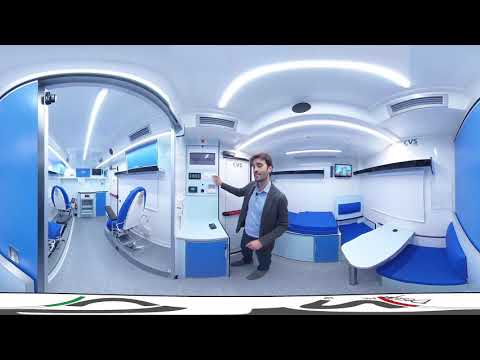This is an image of a brightly lit, white room resembling a laboratory or medical clinic, possibly captured with a GoPro, given the slight distortion and cylindrical perspective. The central figure is a Caucasian male in his mid-30s, with dark brown, almost black hair and fair skin. He is wearing a light blue, collared button-down shirt under a gray business suit jacket, paired with dark pants and gray shoes. The man is standing near a control panel mounted on the wall, pressing its buttons, seemingly demonstrating or operating the device. 

The room features bright blue accents, including a prominent blue gurney and matching blue chairs, which contribute to the clinical and refreshing decor. The space is equipped with various devices, including a small monitor on the wall, and is well-lit by fluorescent lights. The walls are predominantly white with hints of blue, and the room has architectural details such as arched doorways and perhaps a recessed area that holds the blue gurney. The overall setting, compact and bustling with equipment, suggests a specialized use, likely for medical or scientific purposes.